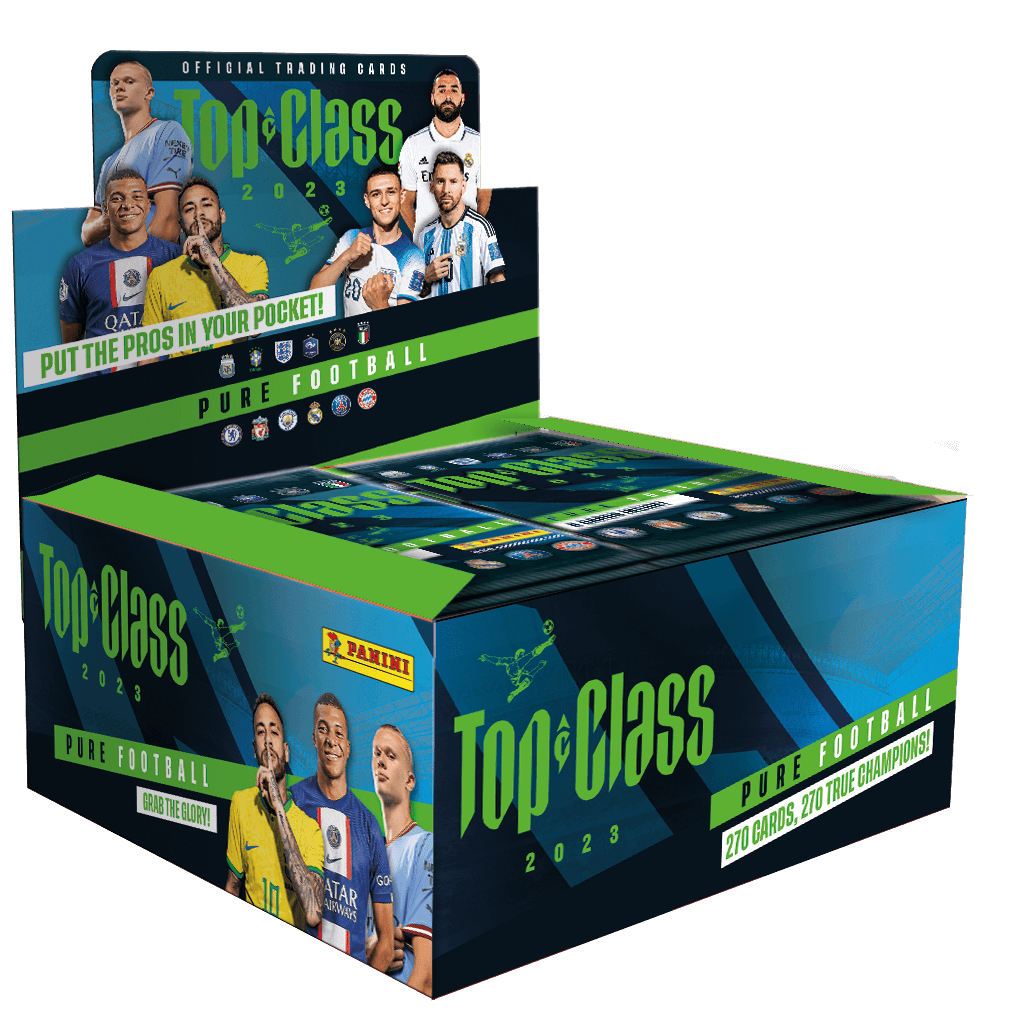The photograph showcases an advertisement for a box of soccer player trading cards. The box features vibrant images of six different soccer players in various uniforms displayed prominently around the main text. The primary title on the box reads "Top Class 2023" in green print, positioned under a label stating "Official Trading Cards" in white text on a black strip. On the top of the box, the slogan "Put the Pros in Your Pocket" is displayed within a white banner in green text. Beneath this, a green bar with black and white typography declares "Pure Football." The front of the box highlights "Top Class 2023, Pure Football, 270 Cards, 270 True Champions" in green print on blue and dark blue backgrounds. The entire box is depicted on a plain white background, providing a clear and focused view of its detailed and colorful design. The box is approximately five inches high and five to six inches wide, shown slightly tilted with the top opened to reveal the blurred fronts of the cards inside.